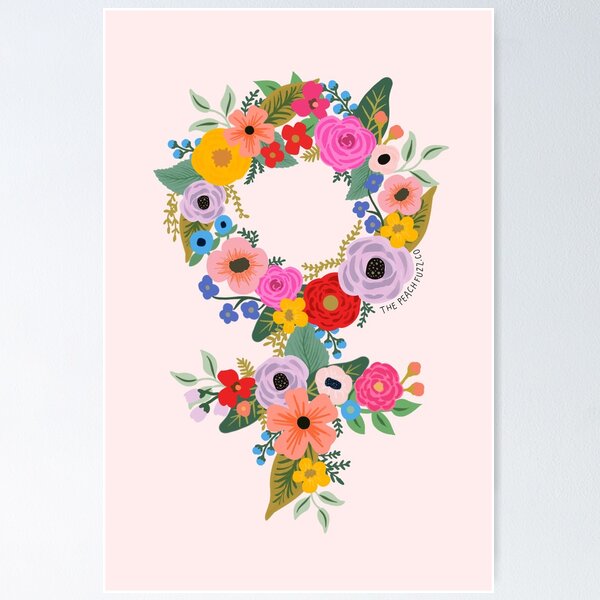The image is a digital illustration that resembles the front of a greeting card. It features a detailed floral arrangement on a pale peach-colored background in a portrait orientation. The main element is a wreath-like ring of flowers composed of bright and pastel-colored blossoms including hot pink, red, lilac, purple, yellow, orange, peach, and blue. Interspersed among the flowers are light and dark green leaves as well as some berries. Below the circular wreath, there is a vertical trailing extension made up of more flowers and greenery, resembling a cross or the female symbol. On the side, near the flowers, is a small tagline that reads "the peachfuzz.co".